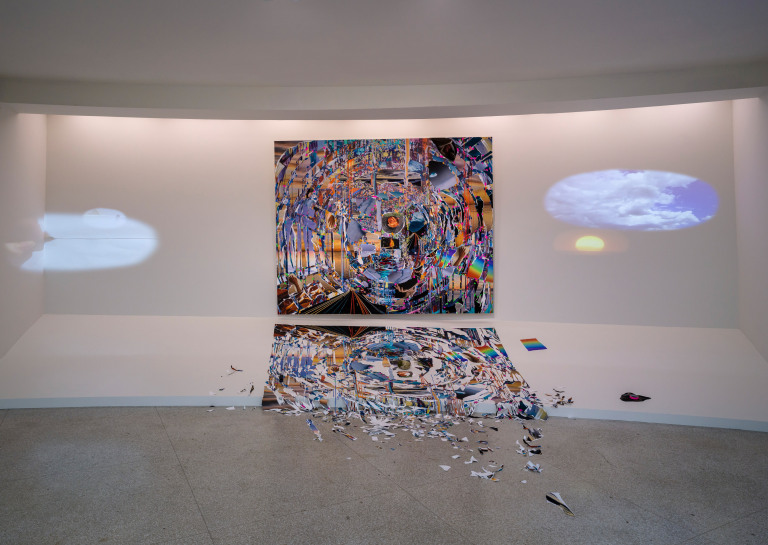The photograph captures an engrossing art display, likely located in a modern gallery space. The installation features a seamless integration of wall and floor, both adorned with the same abstract artwork. This artwork, square in shape, is composed of dynamic drips and diagonal lines in a palette of golds, blues, grays, and blacks. The intriguing part of the display is the continuity of the art piece from the wall to the floor, creating the illusion of a reflection. However, the floor portion of the artwork seems fragmented and dispersed into various bits and pieces at its lowest edge. The material of these fragments remains ambiguous, possibly suggesting broken canvas or shattered glass, adding a layer of mystery and depth to the visual experience.